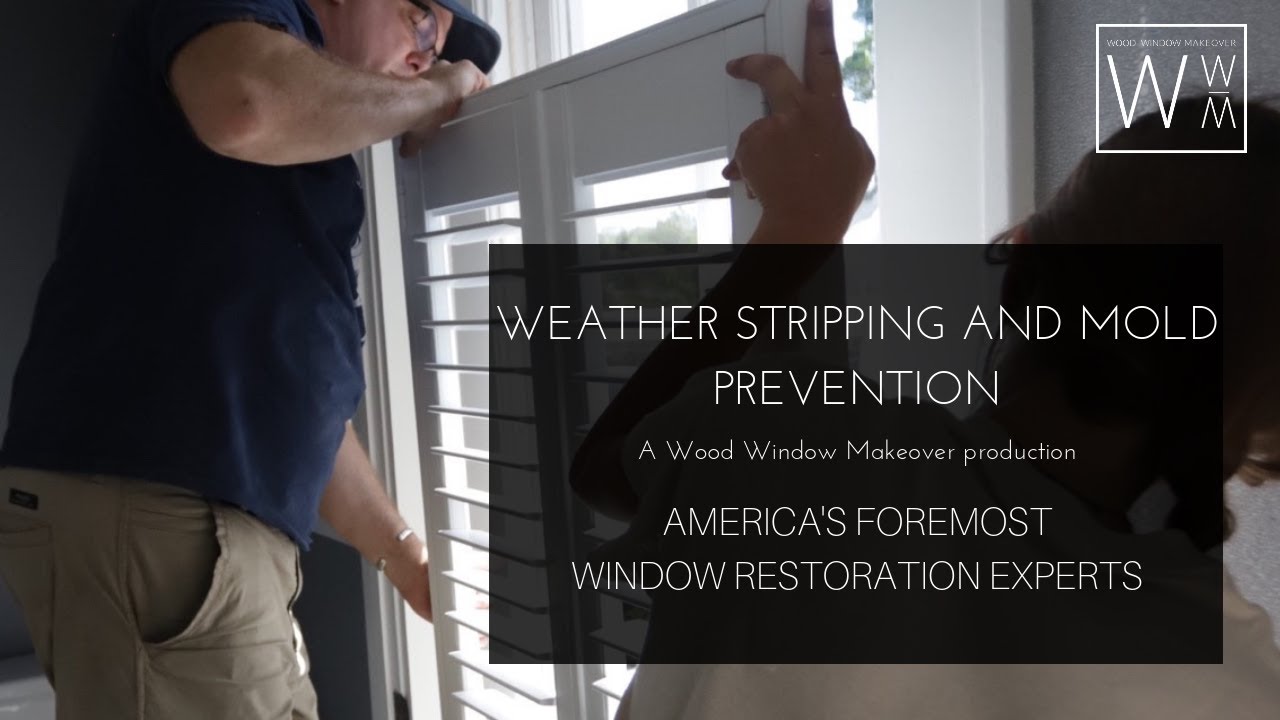The image is a detailed advertisement for "Weather Stripping and Mold Prevention," created by "Wood Window Makeover Production," touted as "America's Foremost Window Restoration Experts." The photo prominently features two workmen installing wooden blinds on a window. One man, wearing a blue cap, blue polo shirt, and tan pants, is clearly visible, while the other is partially obscured behind promotional text. The second man, also in khaki attire, assists in the installation. The scene is overlaid with a black rectangle bearing white text detailing the services offered. Additionally, the upper right corner of the advertisement features a logo showcasing a white square with a capital 'W' next to a smaller 'W' and an inverted 'W' shaped like an 'M'. The overall setup suggests the image could also serve as a cover for a manual or a section of a website dedicated to these specialized window treatments.